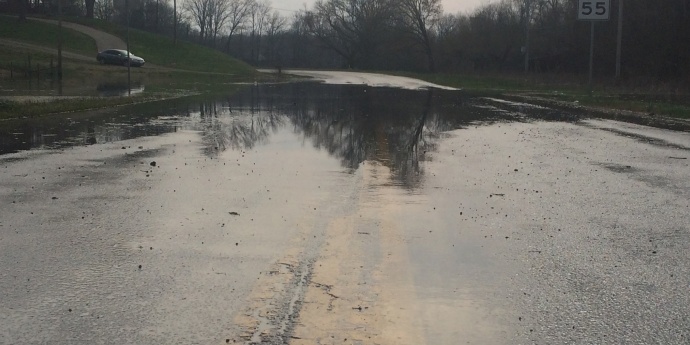In this detailed photograph, taken low to the ground on a grey, overcast winter day, we see a rural road heavily flooded by a large puddle that stretches from the left side to the right, deeply submerging the yellow center lines. The reflective surface of the water mirrors the surrounding area. In the distance, a lonely car can be seen on a section of the road that winds up a small hill and loops around. Grass lines both sides of the road, leading up to areas where leafless trees stand in a dense forest. A 55 mph speed limit sign is prominently visible on the far right, close to more grass and a curb. The grey, cloudy sky overhead adds to the somber and serene atmosphere of the scene.